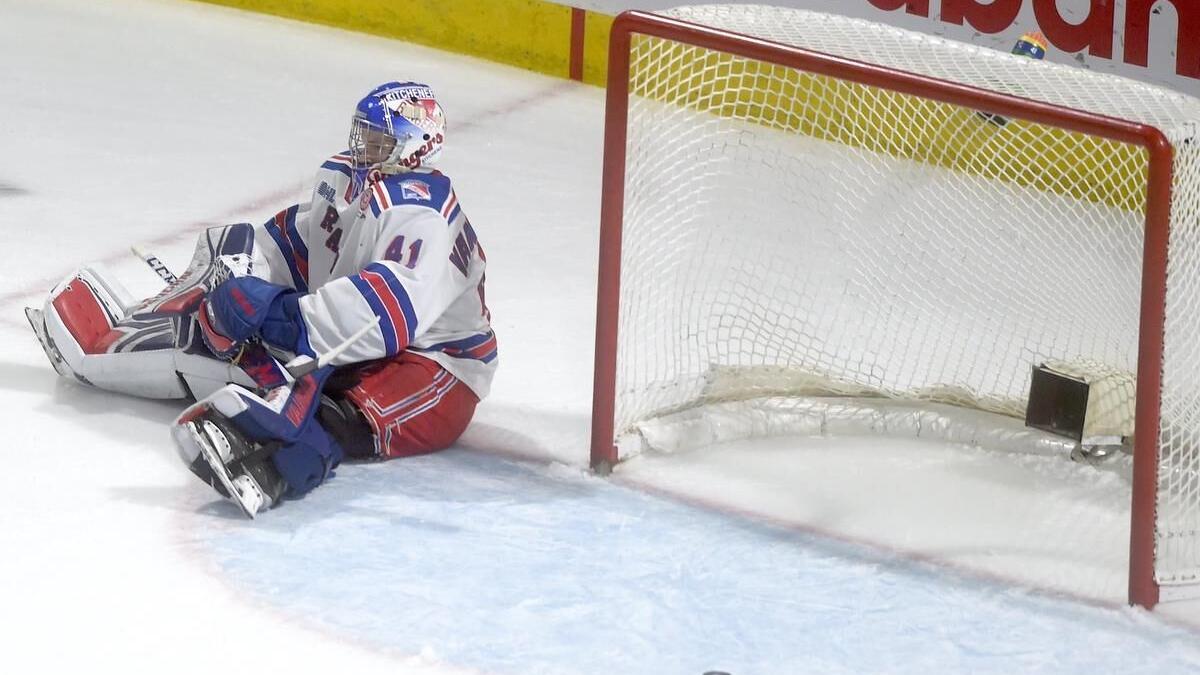This photograph captures a dramatic hockey scene featuring a Texas Rangers goalie, identifiable by the number 41 on his red, white, and blue uniform. The goalie, adorned in a blue, red, and white helmet, is seated directly on the ice beside the left of the red goal post with white netting. His legs are spread in a V shape with blue boots pointed outward, highlighting the wear and tear of the ice, indicative of an intense game. The uniform details are precise: blue over the shoulders, red and blue stripes on the elbows, and red pants. Although his face is obscured, the goalie appears to be holding an indistinguishable object in his hand, suggesting the photo was captured mid-action, possibly following a fall or injury. The scene embodies a moment of pause amidst the brisk pace of the game.